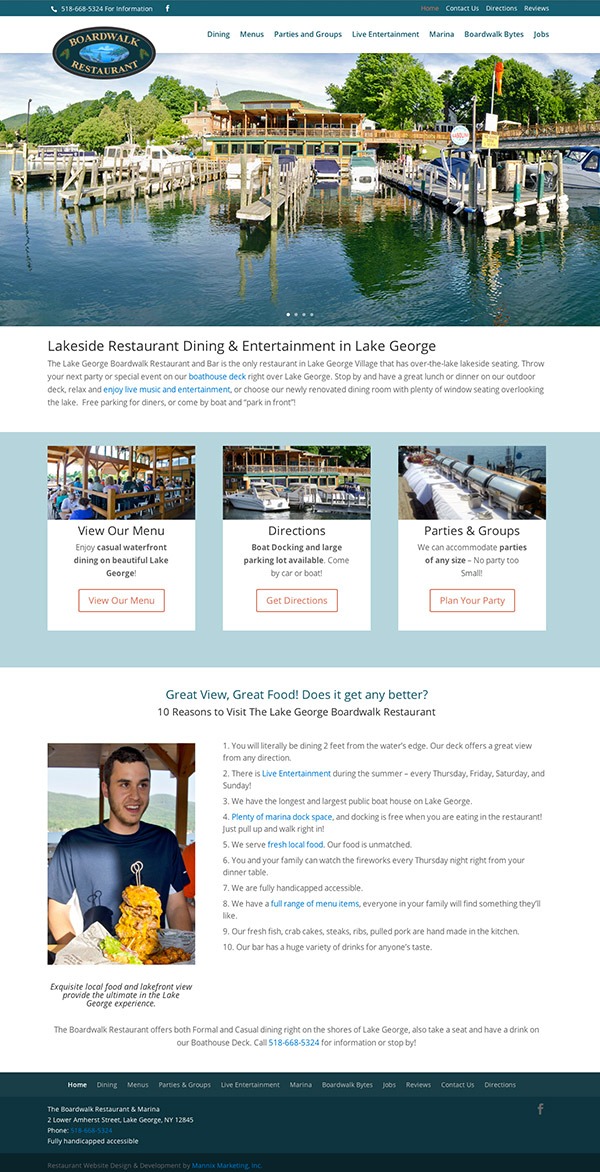The image showcases a picturesque view from the Boardwalk Restaurant at Lake George. In the foreground, several docks stretch along a tranquil waterway, with boats moored alongside, hinting at the bustling yet serene activity of the area. In the background, the restaurant itself is visible, featuring extensive outdoor dining spaces perfect for a meal under the open sky. The setting is framed by lush trees and a vibrant blue sky, creating a scenic and inviting atmosphere. A sign for the Lake George Boardwalk Restaurant and Bar emphasizes its unique offering as the only venue in Lake George Village with lakeside seating. The establishment invites patrons to host parties and special events on their boathouse deck, directly overlooking the lake. Guests are encouraged to stop by for lunch or dinner on the outdoor deck, which boasts live music and entertainment, or to dine in the newly renovated dining room that offers ample window seating with lake views. Convenient parking is available for diners, with the added option of arriving by boat and docking right in front. The promotional message rounds off by highlighting their menu offerings, directions, and event hosting capabilities, all underlined by the tagline: "Great view, great food. Does it get any better?"